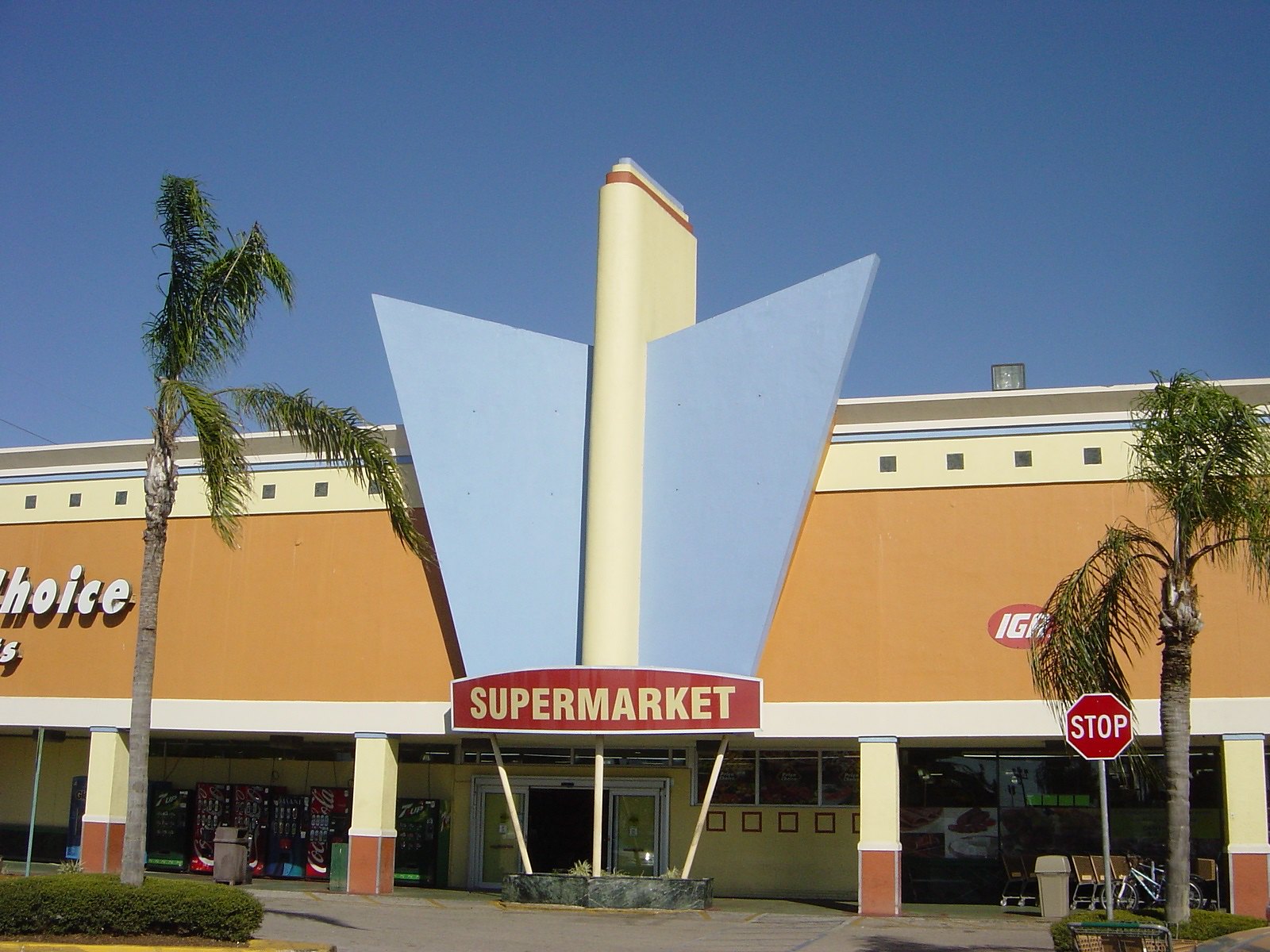In the photograph, we see the front facade of a retro-styled grocery store, distinguished by a prominent marquee featuring two fin-like structures protruding from a central tower. These fins, reminiscent of the tail fins on vintage cars or the back of an arrow, evoke a classic 1950s architectural design. The large sign on the marquee proudly displays the word "Supermarket." Flanked by gracefully arching palm trees, this scene suggests a location in either Florida or California. The winged tower, supported by several poles, adds to the nostalgic charm of the building. In the foreground, a stop sign indicates that the photo was taken from the vantage point of the parking lot, offering a comprehensive view of this stylish and uniquely designed grocery store.